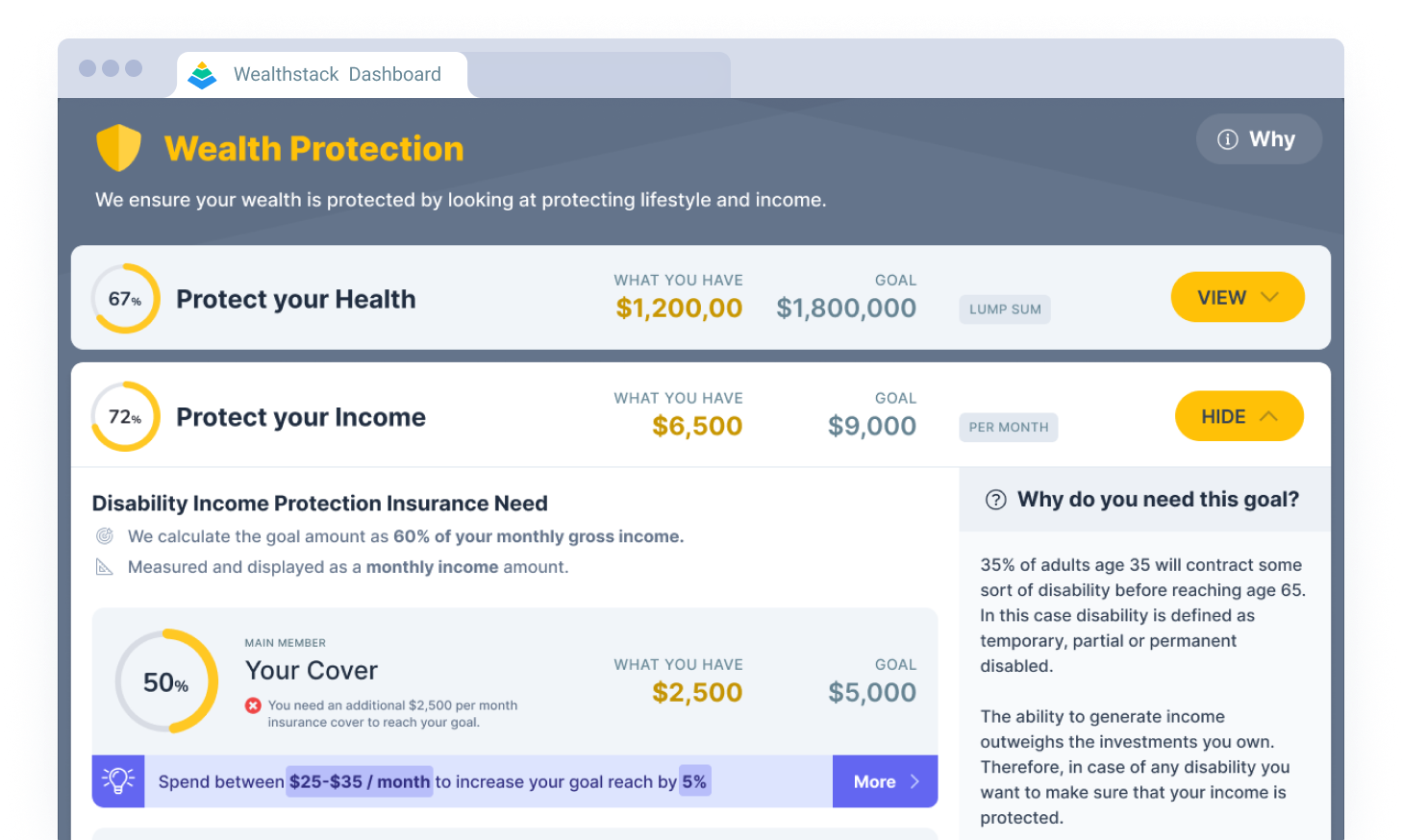Screenshot of a Mac web browser displaying the Wealthstack Dashboard. The browser interface is identifiable by the trio of colored circles—red for closing, yellow for minimizing, and green for expanding—situated in the top left corner. The active tab is white, labeled "Wealthstack Dashboard," and accompanied by a small icon to the left; other tabs appear in gray.

The webpage itself features a dark gray background. Positioned at the top is a yellow heading with the text "Wealth Protection," paired with a shield icon to the left. Just below, a prominent white heading reads, "We ensure your wealth is protected by looking at protecting lifestyle and income." A "Y" button, displayed in white, occupies the top right corner of the screen.

The central section of the dashboard is populated with various metrics displayed in gray, yellow, and white backgrounds. One key metric, labeled "Protect Your Health," reveals that the user has accumulated $1.2 million towards a goal of $1.8 million, achieving 67% of the target. A yellow "View" button alongside allows for data expansion. Another expanded metric, "Protect Your Income," indicates that the user has reached 72% of their goal.